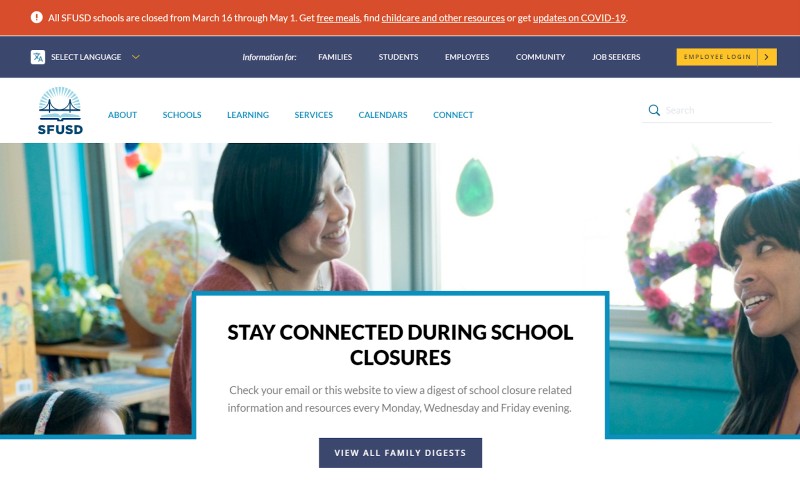The image is a detailed, multi-sectioned announcement regarding school closures and available resources. 

At the top of the image, there is a red banner featuring a white circle with a red exclamation point. Inside the banner, white text reads: "All SFUSD schools are closed from March 16th through May 1st."

Below this, there is further information in white text on a blue background, offering guidance on obtaining free meals, child care, and other resources, along with updates on COVID-19. The text directs readers to "select language," "information for families," "students," "employees," "community," and "job seekers."

Following this, within a yellow rectangle, black text reads: "Employee login," accompanied by an arrow pointing to the right.

The background then changes to white and includes headers such as "About Schools," "Learning Services," "Calendars," and "Connect." A search box, faint gray with a magnifying glass icon and the word "search" underlined in gray, is positioned nearby.

In the image, there are two women and a young girl. One woman appears to be Asian with black hair cut at her chin. The other has black bangs and may be Hispanic or Indian. The girl, partially visible, has a white headband with pink coloring. In the classroom setting, a globe, flowers, desks, windows, and a peace sign made out of flowers are visible.

Finally, black text on the image advises: "Stay connected during school closures. Check your email or this website to view a digest of school closure-related information and resources every Monday, Wednesday, and Friday evening."